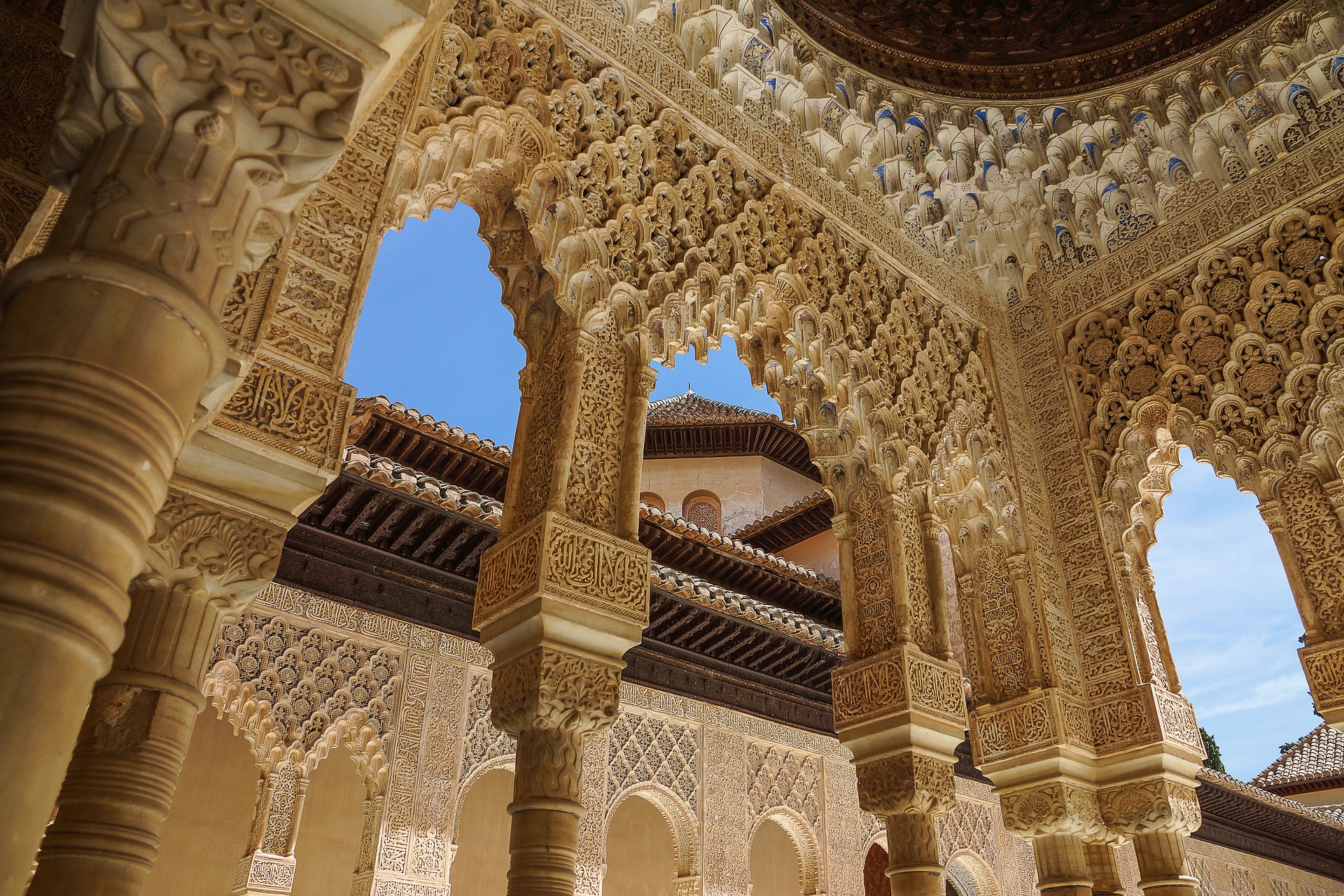This is a detailed landscape photograph of the Alhambra, a historic Nasrid palace located in Granada, typifying Moorish culture. The image captures a striking upward view from the ground level into the intricate ceiling of an open-air section of the palace. The ornate ceiling features elaborate carvings and detailed artistry, highlighted by pointed Moroccan-style arches made of goldish or sandstone-colored stone. These arches, standing on carved columns, open out to reveal a beautifully clear blue sky and a turret from another building in the background. Some walls in the image meet to form a corner under a partially visible dark bronze dome with floral and illustrative designs. The adjacent building visible through the arches exhibits similar detailed carvings and ornate arches, contributing to the palatial and medieval architectural splendor captured in this photograph.